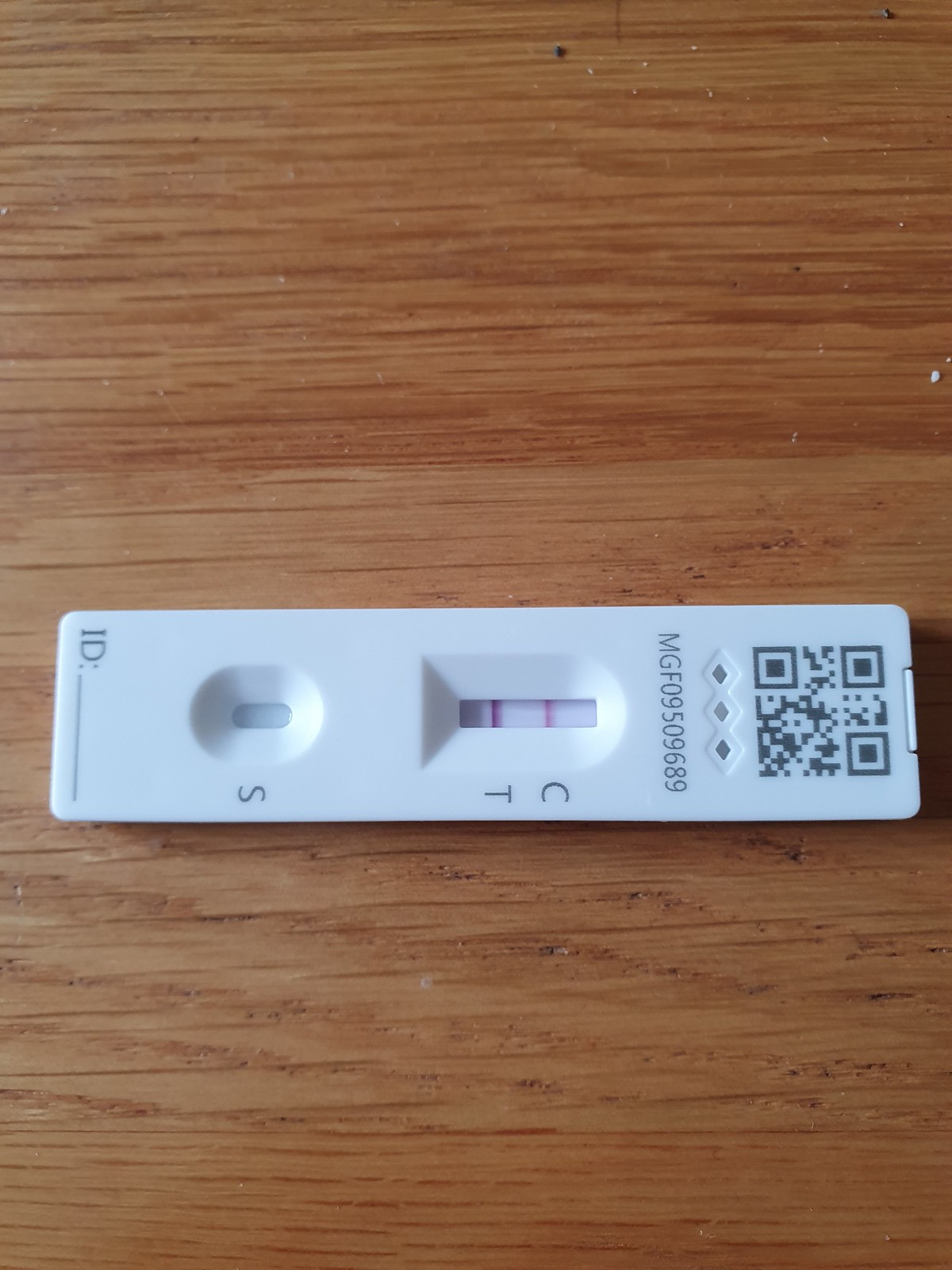The image depicts a COVID-19 test kit placed on a wooden table with a horizontal wood grain pattern. The test kit is positioned sideways, oriented so that it faces to the right. The test kit features a white background. At the top, there is a QR code, which can be scanned for more information. Below the QR code is a sequence of characters: MGF09509689, with three diamonds separating the numbers and the QR code. Further below, there are the letters "C" and "T" with two red lines between them, indicating the test results. Directly to the right of that is a small rectangle containing the letter "S". At the bottom of the test kit, there is an "ID:" label followed by a blank line intended for identification purposes.